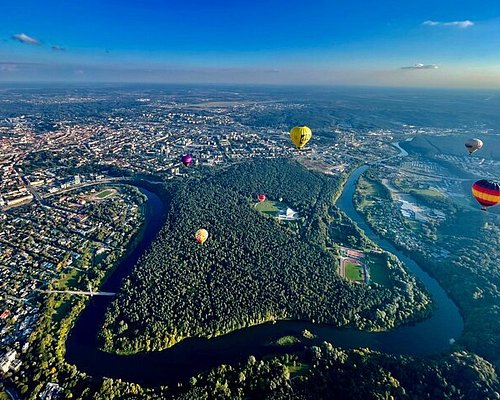This stunning aerial photo captures a lively scene of six vibrant hot air balloons at various stages of flight over a diverse landscape. The photograph, taken presumably from another balloon, showcases a mix of urban and natural elements. Dominating the image, a river winds gracefully from the left, forming a unique W shape before vanishing into the horizon. This river encircles a densely wooded area, creating a quasi-island effect. The surrounding cityscape, primarily concentrated in the left and upper quadrants, contrasts with the lush forests and intermittent clearings, including what appears to be a sports field or stadium.

The sky is a brilliant blue, lightly punctuated by a few white clouds and tinged with subtle purple hues. The sun can be seen setting in the distance, adding a golden glow to the scene. The six hot air balloons, each distinct in color, dot the sky and ground, adding splashes of red, yellow, purple, black, maroon, and white. Notably, a prominent yellow balloon sits centrally, capturing immediate attention, while another balloon with blue, red, and yellow stripes is spotted toward the right. Though buildings and houses are visible below, they are too small to discern specific details, giving an impression of the vast scale of this breathtaking aerial vista.